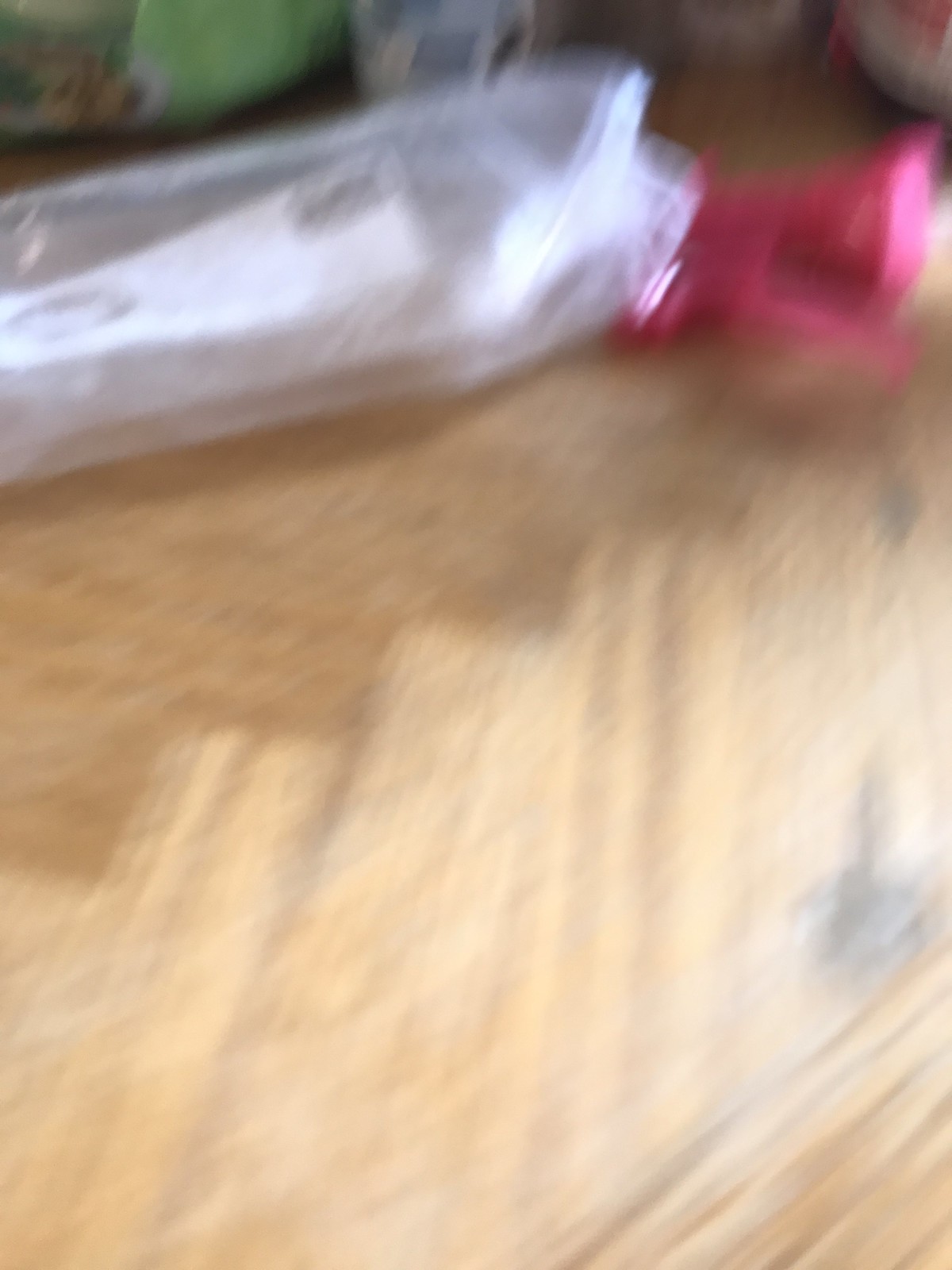A blurry photograph captured at hip height inside a kitchen shows a wooden cutting board on a countertop. On the cutting board, there is a plastic bag, and in the background, a vegetable is partially visible. The image seems to have been taken unintentionally, likely when someone was pulling their phone out of their pocket and accidentally snapping a picture. The scene is cluttered and unfocused, giving the impression of a momentary, candid glimpse of kitchen prep.